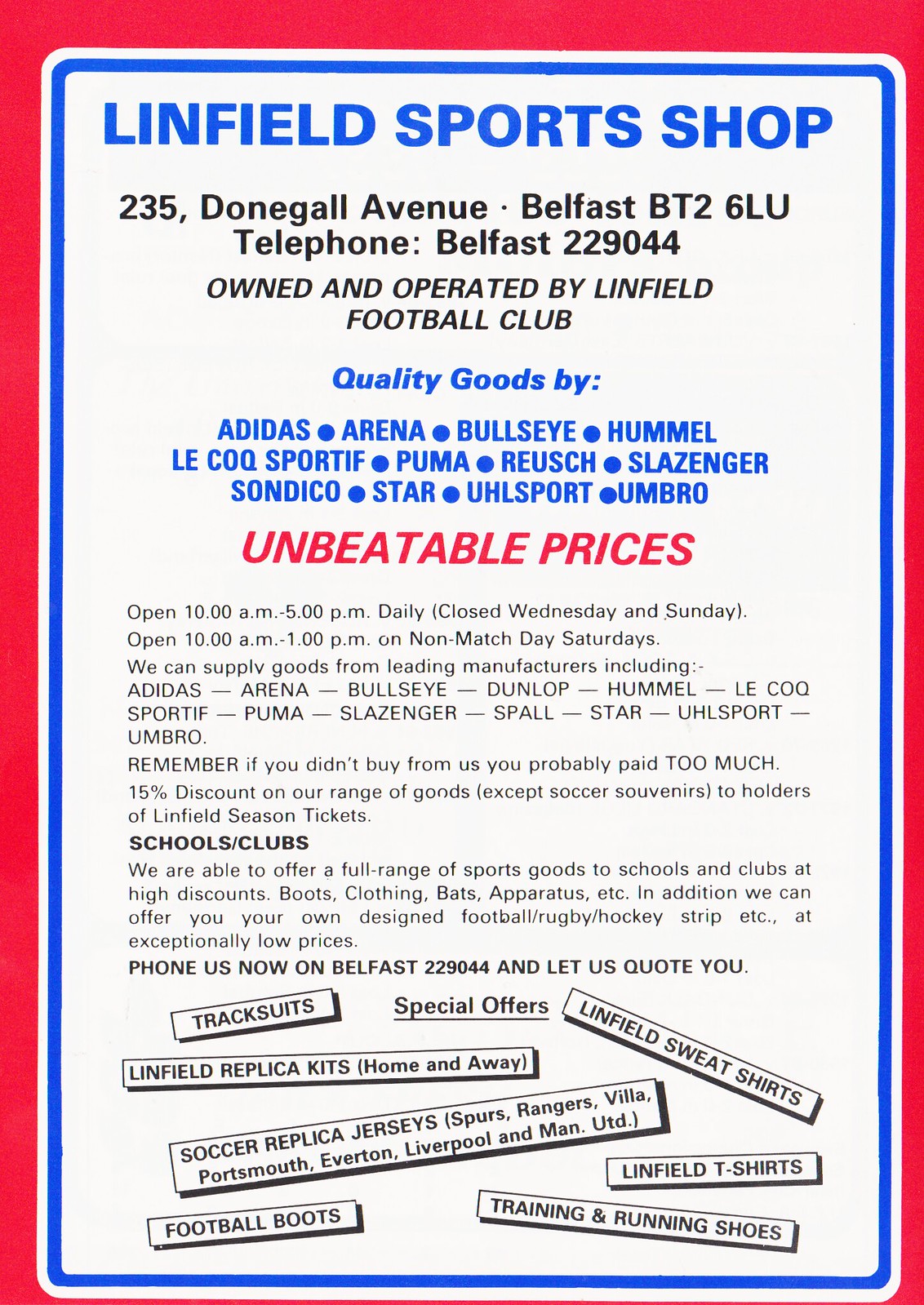The promotional flyer for Linfield Sports Shop features a striking design with a solid red border, followed by a thinner white border, and then a blue border framing the entire image. At the very top, in light blue text, reads "Linfield Sports Shop." Below that, in black text, the address and contact details are listed: "235 Donegal Avenue, Belfast BT2 6LU, Telephone: Belfast 229044." It also highlights that the shop is "owned and operated by Linfield Football Club."

The flyer prominently advertises quality goods from a variety of renowned brands in blue text: "Adidas, Arena, Bullseye, Hummel, Le Coq Sportif, Puma, Roosh, Slazinger, Sandico, Star, UHL Sport, Umbro." Following this, in bold red text, it proclaims "Unbeatable Prices."

Further details in black text provide additional information: Store hours, a reminder that if "you didn't buy from us, you probably paid too much," and a special offer of a "15% discount on our range of goods (except soccer souvenirs) to holders of Linfield season tickets." The flyer also mentions their participation with various schools and clubs, able to offer a full range of sports goods at high discounts, including boots, clothing, bats, and apparatus.

A special section outlines that the shop can supply customized sports gear for football, rugby, hockey, and more at exceptionally low prices. It encourages potential customers to "Phone us now on Belfast 229044 and let us quote you."

Additionally, special offers are highlighted in small text boxes at different angles along the bottom of the page, listing items like track suits, Linfield t-shirts, and training and running shoes. The fonts throughout are a mix of blue, black, and red on a white background, enhancing the visual appeal and readability of the flyer.